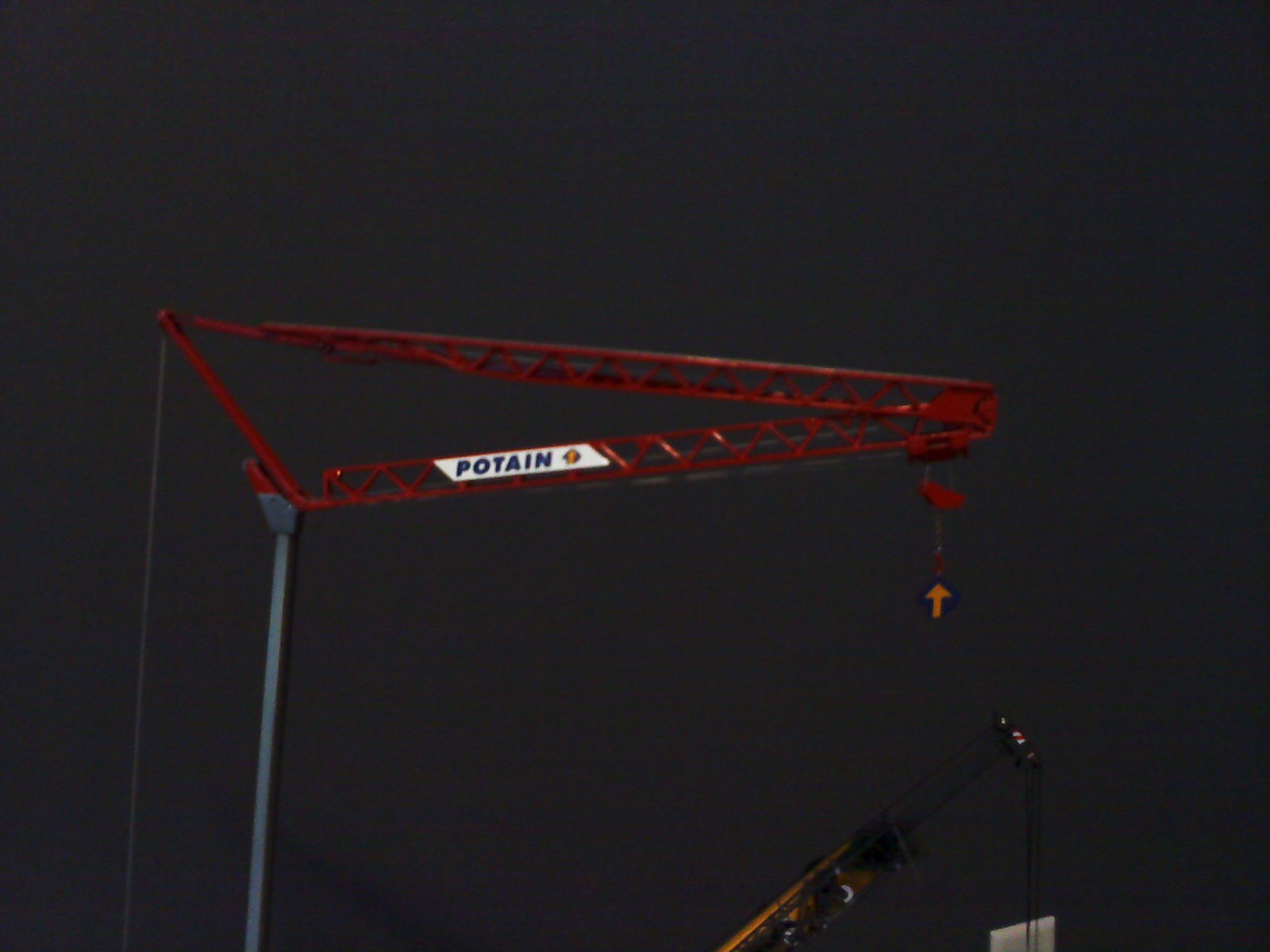This color photograph, taken at night against a nearly black sky, captures the top portion of a steel crane. The crane is supported by silver posts and features a prominent, red, triangular-shaped arm extending from the left to the right of the image. The arm, which narrows to a point on the right side, has a white sign with the word "POTAIN" written in navy blue, all-capital letters. Hanging from the pointed end of the crane is an orange arrow, suspended by a chain and pointing upward. Below the arrow, the shadowy outline of another crane is barely visible in the darkness. The photograph, presented in a landscape orientation, showcases detailed realism and highlights the crane's distinct structure against the night sky.